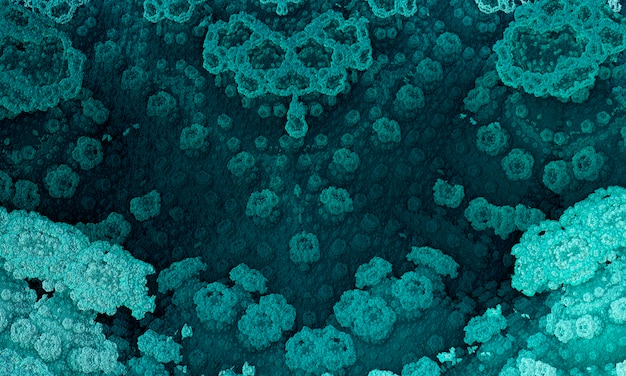The photograph showcases a textured growth with an intriguing pattern and color palette that invites multiple interpretations. Dominated by shades of dark green, light seafoam green, light blue, and white, the irregular shapes and formations create an almost crystalline or coral-like appearance. The growth appears in varied arrangements, some forming circular clusters while others extend in linear patterns, spread across what could be a marine environment, under a microscope, or even on the side of a submerged ship. The formation, partly resembling a V shape with hollowed sections and almost kidney bean shapes, suggests the complexity and organic nature of this subject. The overall texture looks rough, with some parts seemingly soft and delicate, as if entrapped in ice or viewed under magnification. Its abstract nature blends scientific intrigue with artistic allure, leaving one to ponder whether it's a close-up of biological matter or an artist's representation of marine life.